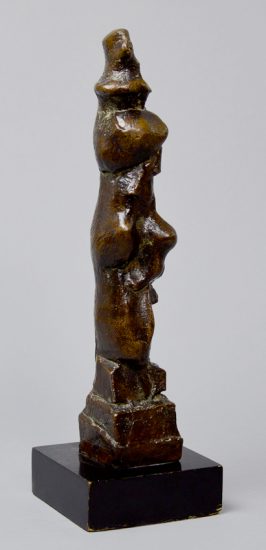This photograph captures a small, intricate bronze statuette with a smooth, dark brown finish adorned with various dark gray spots. The statuette appears to represent three abstract human-like figures stacked vertically, each holding the other up, with the bottom figure seated on a square-shaped, brown throne. It is placed atop a chipped black cuboidal base, revealing a tan underlayer. The image, taken in portrait orientation, is set against a seamless, solid white background with a flat shadow to the right, indicating the light source comes from the left. The sculpted figures rise approximately 14 inches high, mounted on a base about three inches square. The indistinct forms and shiny portions reflect a unique play of light, leaving an impression of a purposeful yet abstract design.